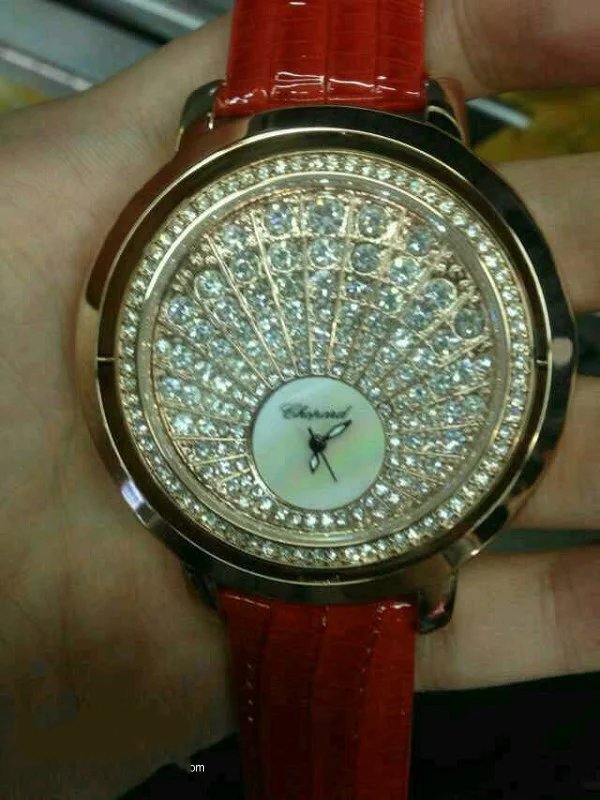This close-up photograph features a woman's hand, with her palm facing up, holding a luxurious and elaborate wristwatch. The watch boasts a shiny gold case adorned with an intricate design of sparkling diamonds or rhinestones that cover almost the entire watch face. At the center of this dazzling display is a small, circular clock face made of Mother of Pearl, without numbers and featuring a pair of delicate Mother of Pearl arrow-shaped hour and minute hands. The cursive logo is written on the clock face, though it's too small and blurry to discern clearly. The watch is paired with a striking red leather or pleather band that mimics reptile skin, adding to the watch’s high-end appearance. The background of the image transitions from black at the bottom to silver and yellow at the top, enhancing the watch's opulence.